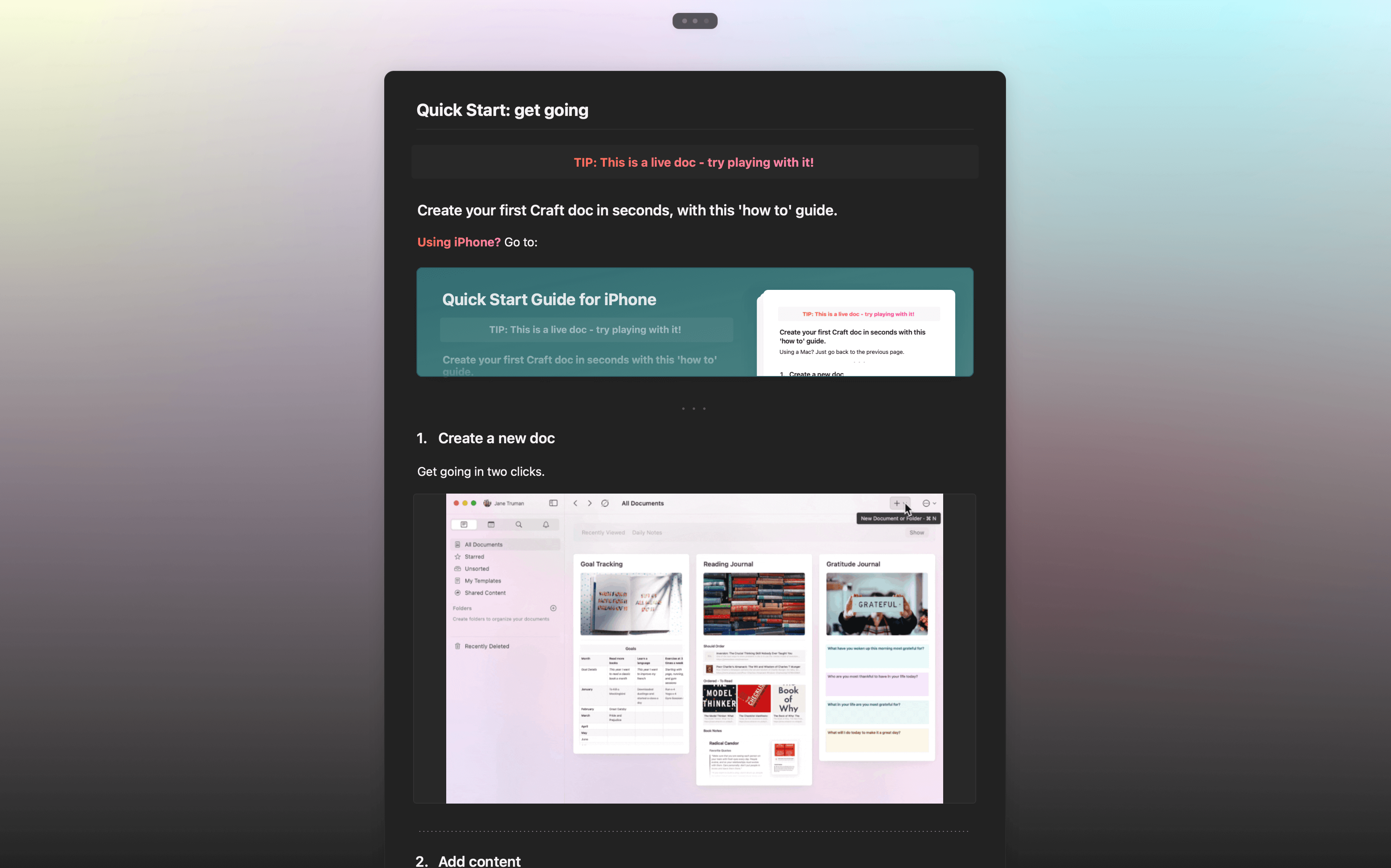The image features a predominantly black background with various visual elements and text overlays. At the center lies a prominent black square. Surrounding this is a backdrop in hues of purple, dark gray, yellow, and blue, creating a visually striking contrast.

At the top of the image, a long rectangular element contains three dots. The text within this rectangle is colored in red and white. The white text says "Quick Start: Get Going," and adjacent red text states "Tip: This is a live craft doc, try playing with it." Further instructions in white text read, "Create your first craft doc in seconds with this how-to guide." Below this, in red, it asks, "Are you using an iPhone?" followed by a prompt in white: "Go to," next to a green rectangular button labeled "Quick Start Guide for iPhone."

The image also includes a step-by-step guide to creating a new document, beginning with "1. Create a New Doc." It encourages users to "Get going in two clicks." Additionally, it shows various document-related elements, such as "Your Documents," "Your Templates," and "Stored" items, along with this person's name in the top corner. An arrow points to a plus sign for creating new documents. Examples of document types, like "Tracking," "Reading Journal," and "Gratitude Journal," are shown on a predominantly white background near the bottom.